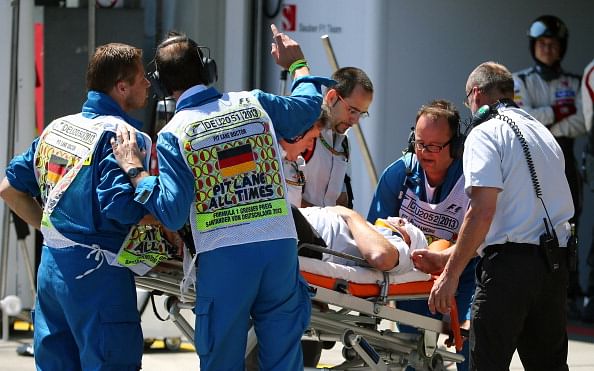In this horizontally aligned rectangular outdoor image, various men surround another man lying on a metallic stretcher with a white cushion. The man on the stretcher, dressed in a white T-shirt and black pants, has his hand resting on his stomach, and it appears he has a bandage around his head and possibly a neck brace. Several individuals, at least six, are tending to him, with particular attention from two men in blue jumpsuits and white vests marked "Pit Lane All Times." These men appear to be part of a race team, indicating this might be a scene from a racing event. Among those gathered, one man stands out in a white polo shirt and black pants, equipped with a walkie-talkie. Additionally, on the upper right side, against a white wall, a figure with folded arms, still wearing a racing helmet, observes the situation. This figure, alongside another partially visible individual in racing attire, underscores the racing context of the image.